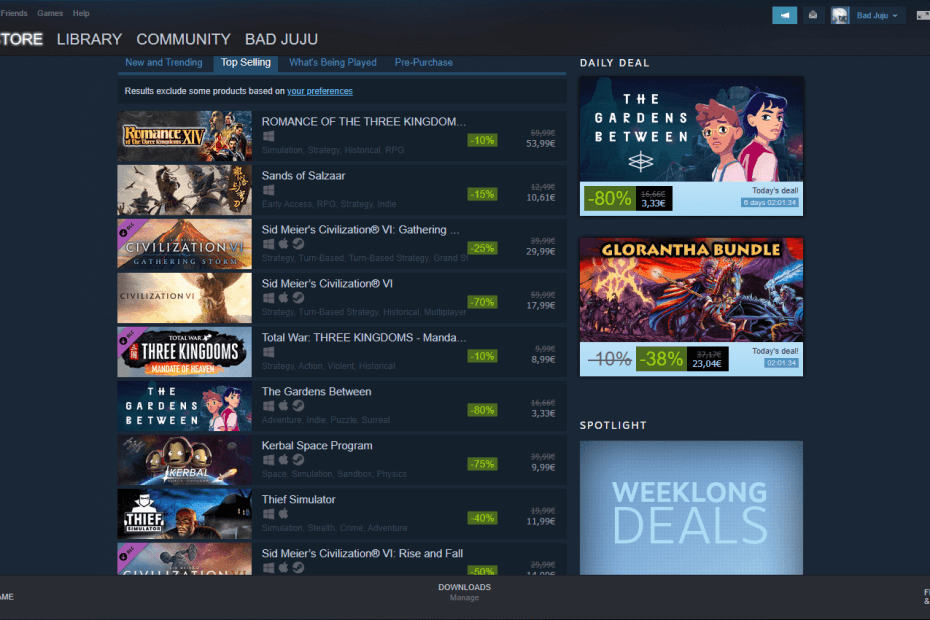The image showcases an organized layout of a digital storefront against a dark blue background. At the top, there are small, indistinct headers. Below them, prominent tabs for "Store," "Library," "Community," and "Bad Juju" are visible. On the right side, there's a conspicuous blue button with a white icon inside.

Highlighted sections include categories such as "New and Trending," "Top Selling" (outlined in white), "What's Being Played," "Pre-Purchase," and "Daily Deal" on the right-hand side. A blue line separates sections, accompanied by white text and underlined blue hyperlinks.

The left side displays various game listings with detailed descriptions:
1. **Romance of the Three Kingdoms** - Accompanied by four small icons, a yellow box indicating "-10%," although the price is hard to discern.
2. **Sands of Salzaar** - Includes four icons and a yellow box showing "-15%".
3. **Sid Meier's Civilization VI: Gathering Storm** - Features four icons, a circle with a check mark, and "-25%".
4. **Sid Meier's Civilization VI** - Lists four icons, an Apple logo, a circle with a check mark, and "-70%".
5. **Total War: Three Kingdoms Mandate of Heaven** - Includes four icons and a green box with "-10%".
6. **The Gardens Between** - Displays four icons, an Apple logo, a circle with a check mark, and "-20%".
7. **Kerbal Space Program** - Shows four icons, an Apple logo, a circle with a check mark, and "-75%".
8. **Thief Simulator** - Details four icons, an Apple logo, and "-10%".
9. **Sid Meier's Civilization VI: Rise and Fall** - Includes four icons, an Apple logo, a circle with a check mark, and "-10%".

Additionally, the bottom includes "Domain," listed very small. The right side features "Daily Deal" offerings, such as "The Gardens Between" at "-80%" and a "Glorantha Bundle" at "-38%". In a blue box, "Spotlight Weeklong Deals" catches attention.

This comprehensive layout points users towards current deals, favorite titles, and new trends in the gaming community.